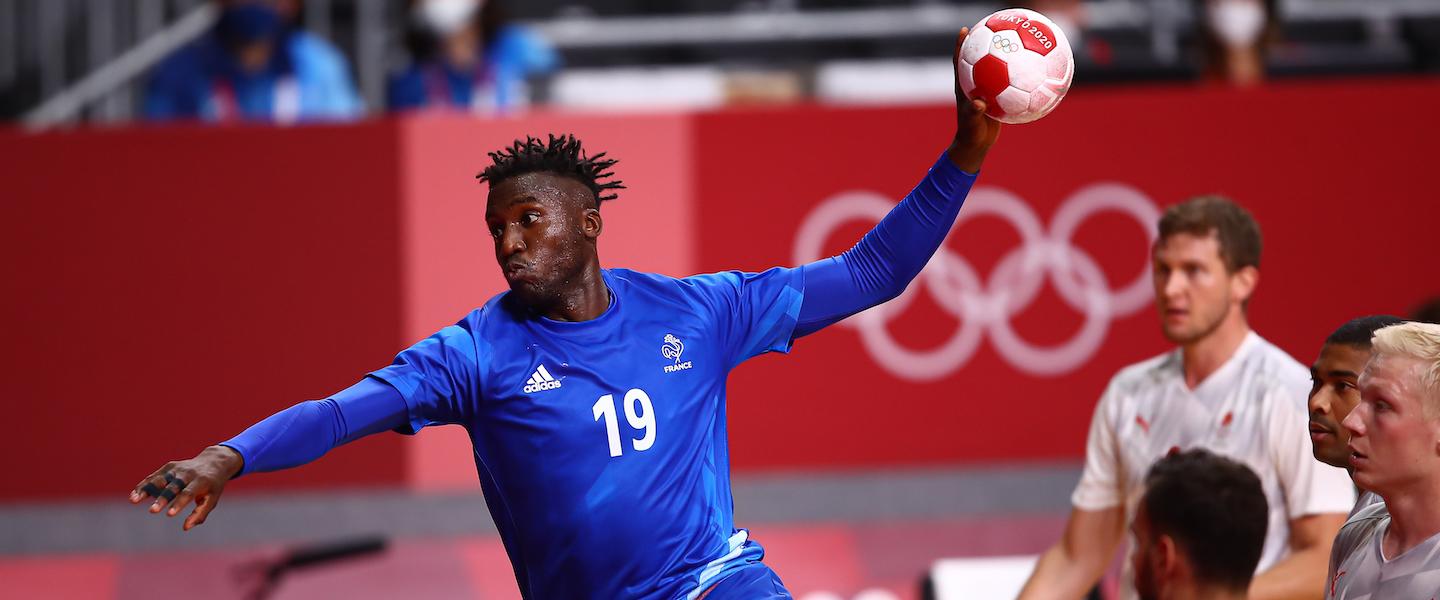A detailed photo captures a tense moment during an Olympic handball game. At the center is a determined player from France, identifiable by his blue Adidas jersey labeled "FRANCE" and his number 19 emblazoned in white. His form is set, as he grips the handball in his left hand, arm pulled back, poised to throw. The white Adidas logo is clear on his chest. In the background, a red barrier prominently features the iconic white Olympic rings, signifying the prestigious setting. The stands behind are filled with spectators, though they appear blurry. To the right side, players from the opposing team sit on the bench, attentively watching the game unfold. Their jerseys are primarily white and grey, accented with touches of red. The scene is tense, with every element indicating the high stakes and intensity of the match.